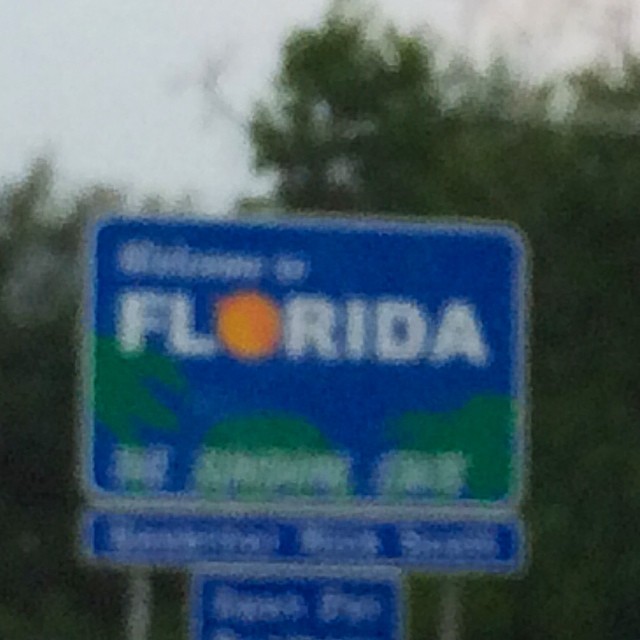The image depicts a rainy scene viewed through a windshield, with raindrops blurring the details. The central focus is a large blue highway sign welcoming drivers to Florida. Despite the blur, the words "Welcome to Florida" are discernible in white letters, with the "O" in Florida creatively depicted as a vibrant orange, highlighting the state's famous citrus fruit. The sign is accented with greenery at the sides and bottom. Below the main welcome message, there are two smaller signs indicating available services, though their exact wording is not clear. The background reveals a dense array of trees, adding to the lush, natural feel of the area.